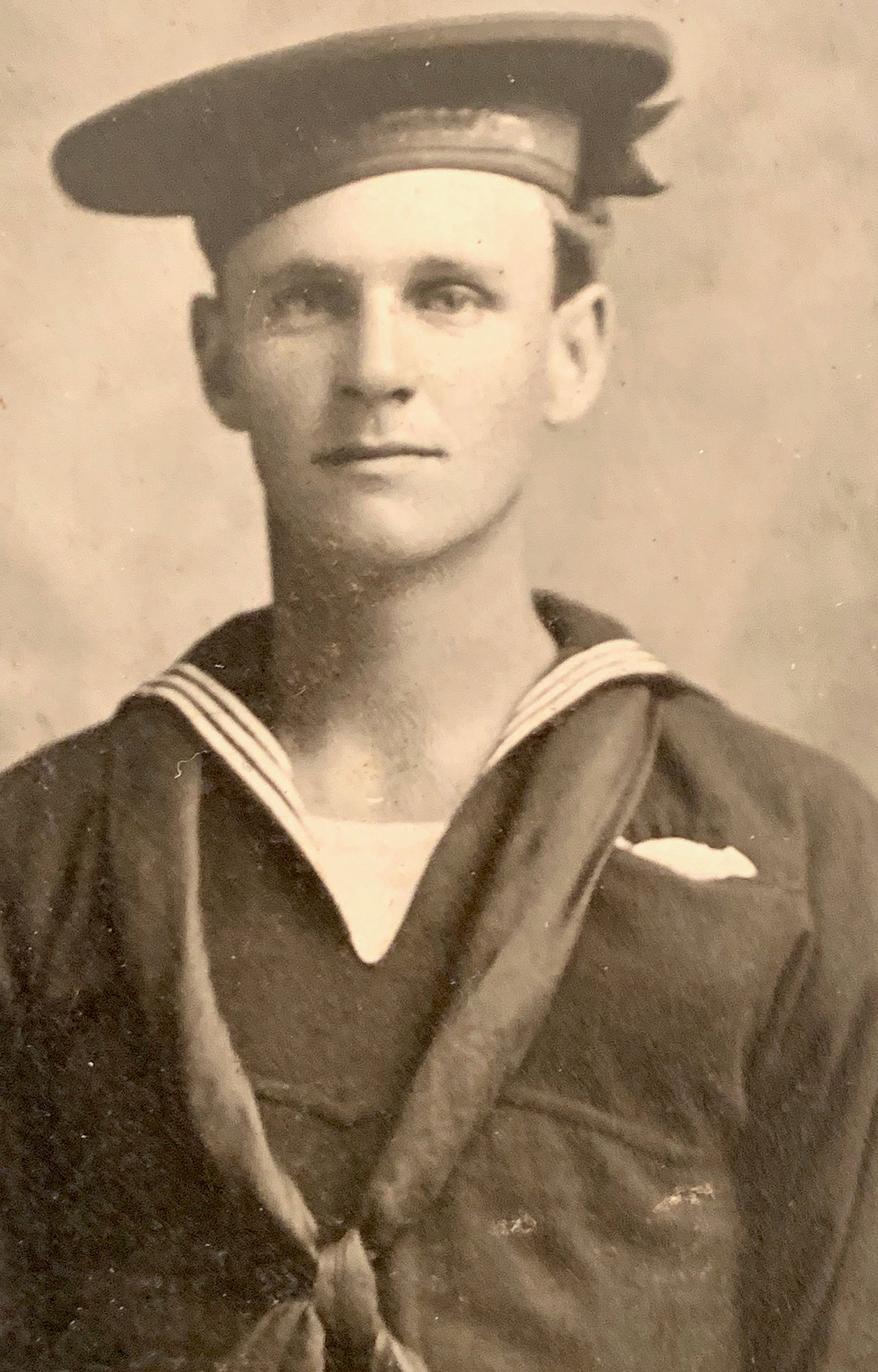This detailed black-and-white photograph, likely taken during the early 1900s to 1920s, captures a young, clean-shaven sailor, who appears to be in his late teens or early twenties. The close-up image, which shows him from the chest up, highlights his distinct sailor or Navy uniform. He wears a traditional sailor cap along with a uniform featuring a V-shaped collar adorned with lines extending outward, a white undershirt, and a tie knotted at the front. Additionally, a handkerchief is tucked into his breast pocket. The portrait, likely taken in a studio setting with a nondescript background, shows the sailor with a slight smile. The photograph itself bears some scuffs and signs of wear, suggesting it is an old family keepsake.